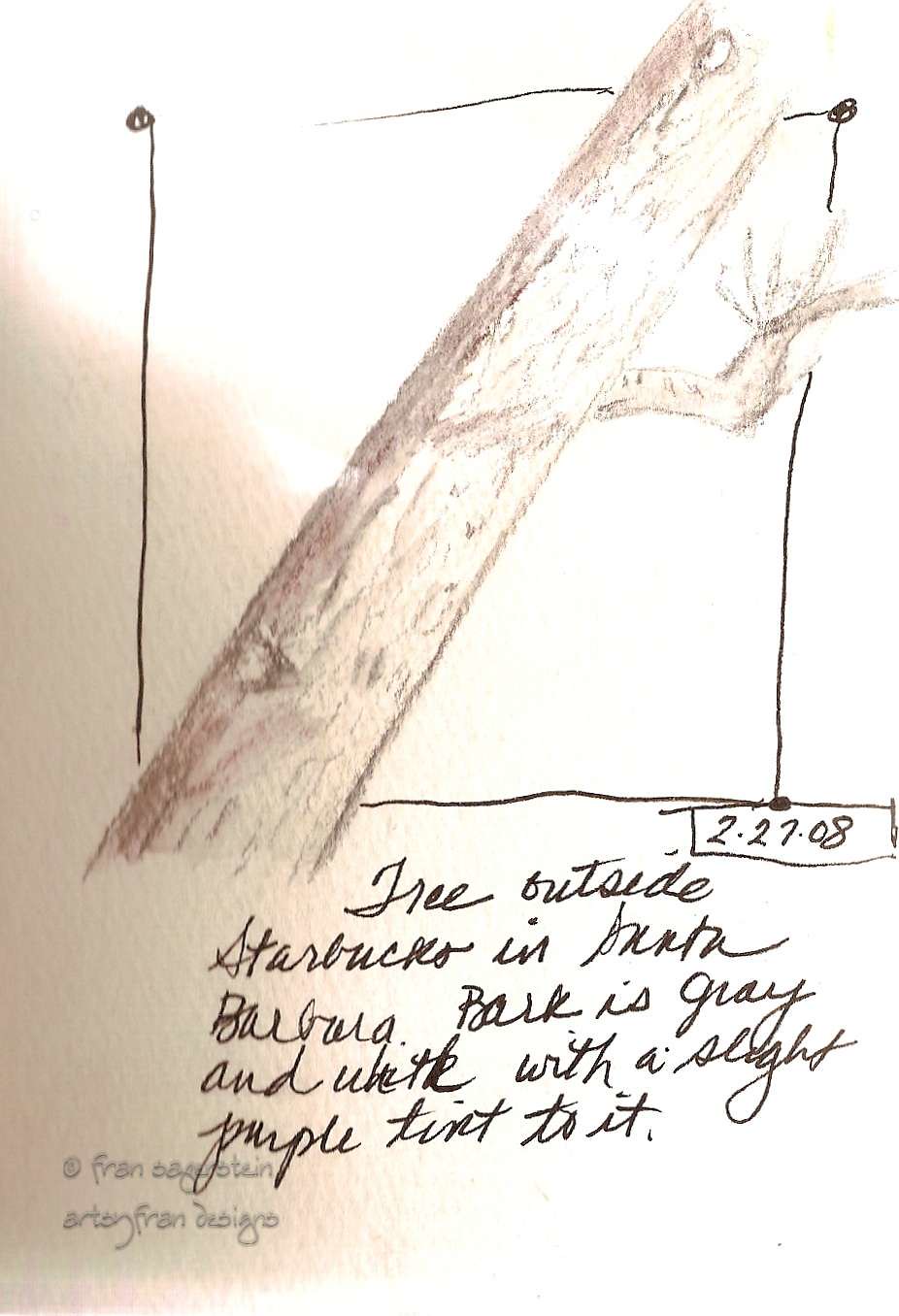This image features a detailed illustration of a tree trunk with a branch extending from the bottom left to the top right corner, possibly created with charcoal or pencil on white paper. A smaller branch juts out to the right side of the main trunk. The illustration is framed by a black pen-drawn border with small circles at each corner. Within the border, there is handwritten text in cursive that reads "Tree outside Starbucks in Santa Barbara. Bark is gray and white with a slight purple tint to it." Additionally, the date "2-27-08" is inscribed in black pen at the bottom right corner of the illustration. Below the date, there is a barely legible watermark that possibly reads "Fran Sebastian and Artsy Fran Designs."